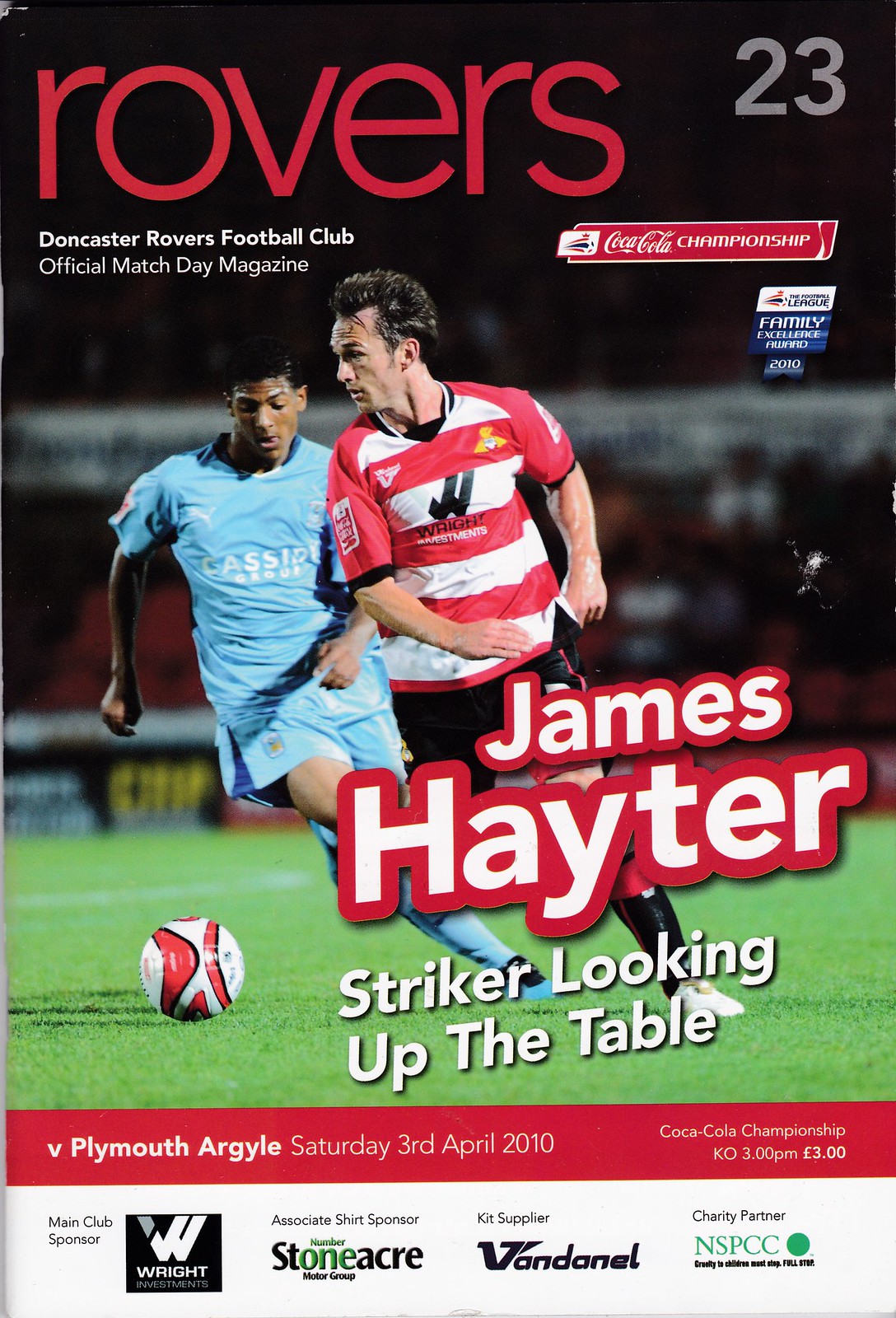The cover of a magazine, titled "ROVERS" in bold red uppercase letters at the top against a black background, with "23" in dark gray on the upper left. Below the title, there's a subtitle in smaller text: "Doncaster Rovers Football Club Official Match Day Magazine." The main image features two athletes in action on a green field, suggesting a soccer match. The foreground shows a white athlete in a red and white striped shirt, black shorts with red accents, black socks with red lines, and white shoes, with a red and white ball nearby. This player, identified as James Hayter, has a stressed expression while leaning sideways, looking both sideways and downward. Behind him is a black athlete in a blue jersey, blue shorts, blue socks, and blue shoes, also leaning sideways in pursuit of the ball. A red bar across the lower portion announces "Plymouth Argyle Saturday 3rd April 2010," with the caption "James Hayter - Striker looking up the table" in large white letters highlighted in red. At the very bottom, sponsor logos for Wright Investments, Stoneacre, Vandernal, and NSPCC are displayed on a white bar with black text.